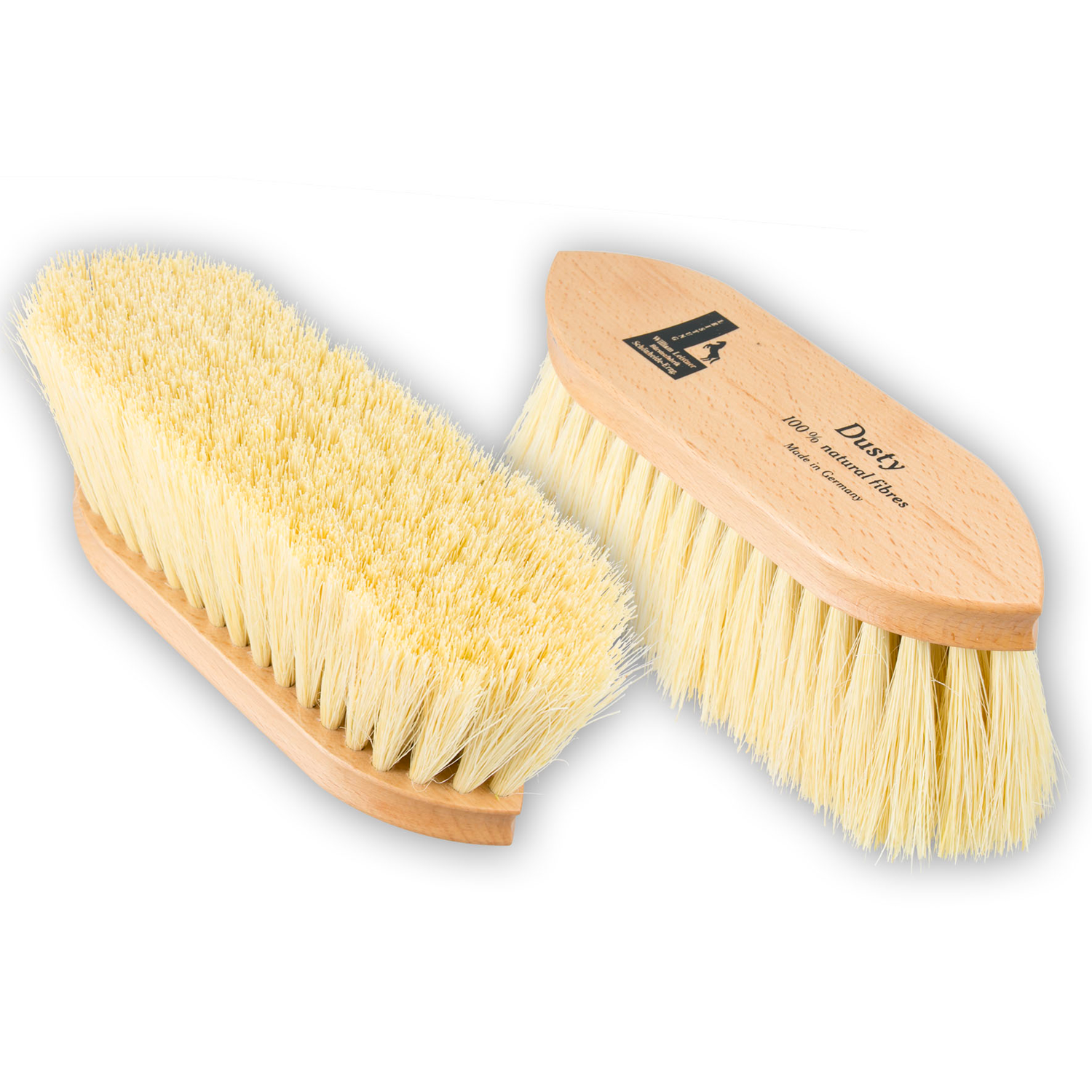This image showcases two horse brushes displayed on a white background. Both brushes feature blonde wood handles and yellow, fibrous bristles made from 100% natural fibers. The brush on the right is oriented to show the handle, which displays an imprint logo of the brand and an image of a horse along with the text "Dusty 100% Natural Fibers, Made in Germany." The brush on the left is flipped to reveal the bristle side, showing densely packed, long, and brittle-looking yellow bristles. The bristles are bound in small bunches and inserted into the wood. The overall design of the brushes is hand-held with an oval-shaped wood top, lacking a separate handle.